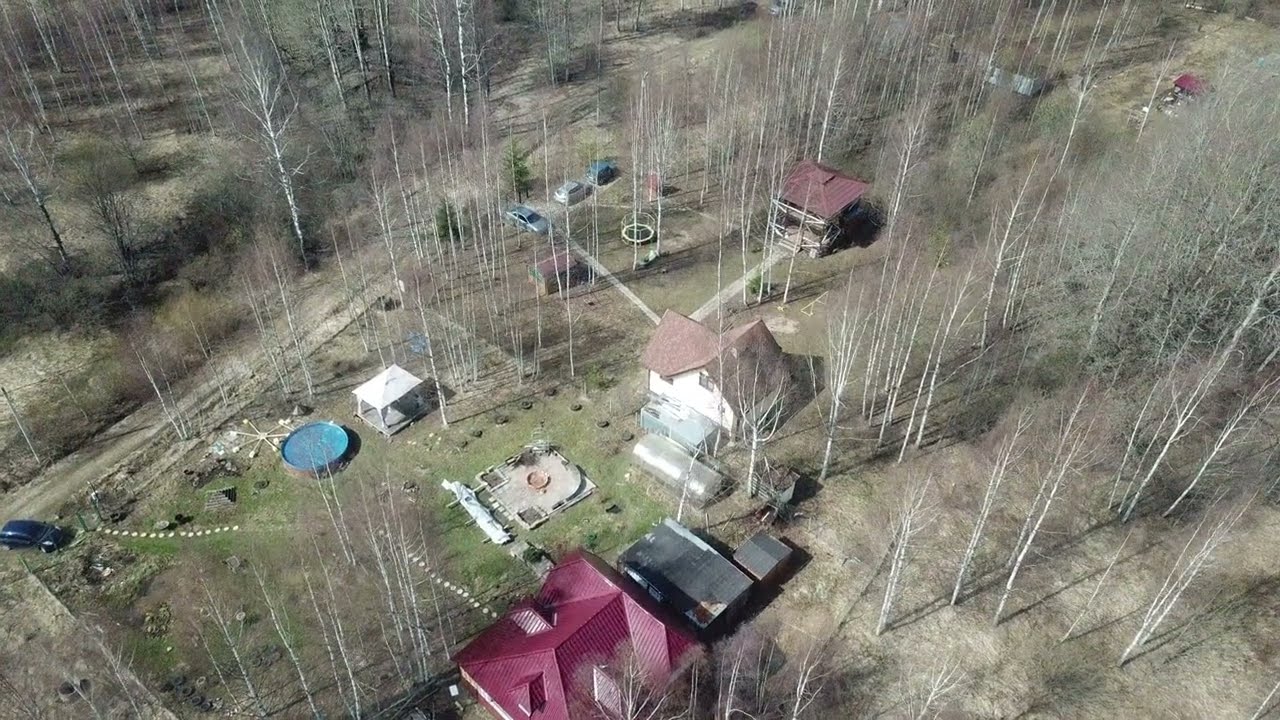This overhead, aerial photograph captures a rural homestead surrounded by a vast landscape of barren, tall trees with white trunks, likely depicting a fall setting. The focal point of the image is a white house with an orange-ish brown roof, situated centrally among several structures. To the right and left of this main house are additional buildings, both with distinct red roofs, and another structure featuring a black roof. There is a cement pad positioned near the center of the property and an above-ground swimming pool or water tank visible to the left. Near the pool, a canopy can be observed, and a trampoline is also present within the property boundaries. The homes appear isolated, far from any town, connected by dirt roads typical of a countryside setting. The area is devoid of people or animals, but a few vehicles are parked in driveways adjacent to the houses. The photograph, bright and clear, shows the entirety of this quiet, rural scene with great detail.